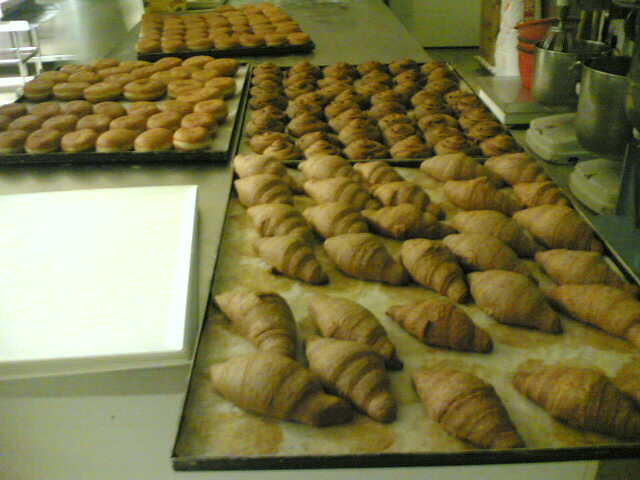This image showcases a bustling bakery kitchen filled with a variety of freshly baked goods. Four large trays dominate the scene, each brimming with delicious pastries and confections. In the foreground, a tray teeming with golden, flaky croissants sits prominently. Behind it, a tray overflowing with perfectly round cinnamon rolls catches the eye, while to the left, another tray is loaded with irresistible glazed doughnuts. Further back, more glazed doughnuts and fruit or cream-filled rolls are neatly arranged. Overseeing this spread, big mixers are perched on a counter above the pastries, ready for the next batch of dough. The stainless steel table they rest on underscores the industrious atmosphere, hinting at the flurry of activity that recently took place. The image is tinged with a slight greenish hue, perhaps due to the lighting, evoking the warm, inviting feel of a dedicated baking space.